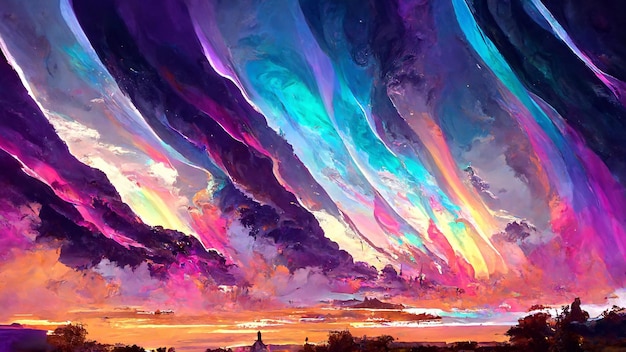This painting depicts a surreal, exterior environment dominated by a vividly multi-colored sky that fills the entire horizon. The sky is composed of ribbons and ripples of various hues including pink, magenta, purple, iridescent white, blue, dark violet, and orange, creating a mesmerizing, almost psychedelic atmosphere. These colors blend and transition into each other, resembling either abstract clouds, smoke, or celestial wisps, making the scene appear trippy and otherworldly. In the background, a church steeple is visible, further grounding the surreal sky in a more tangible landscape. The foreground includes hints of trees and possibly small buildings or islands, adding another layer of depth to the abstract composition.